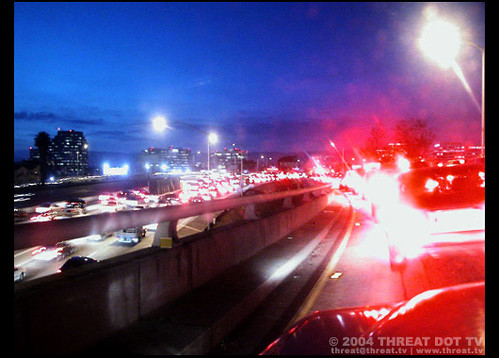The photograph captures a nocturnal outdoor scene. The night sky, a deep shade of dark blue, blankets the top portion of the image, while the presence of car headlights confirms the late hour. On the right side, a road stretches into the background, showcasing the rear ends of several vehicles, their outlines bathed in the glow of red taillights. Opposite this, another road mirrors the same pattern of automobiles, characterized by the distinct red brake lights. In the distance to the left, a large, dark building dominates the horizon, with its windows illuminated, casting a subtle glow against the night. This blend of urban thoroughfare and quiet night sky creates a vivid depiction of a bustling city roadway after dark.